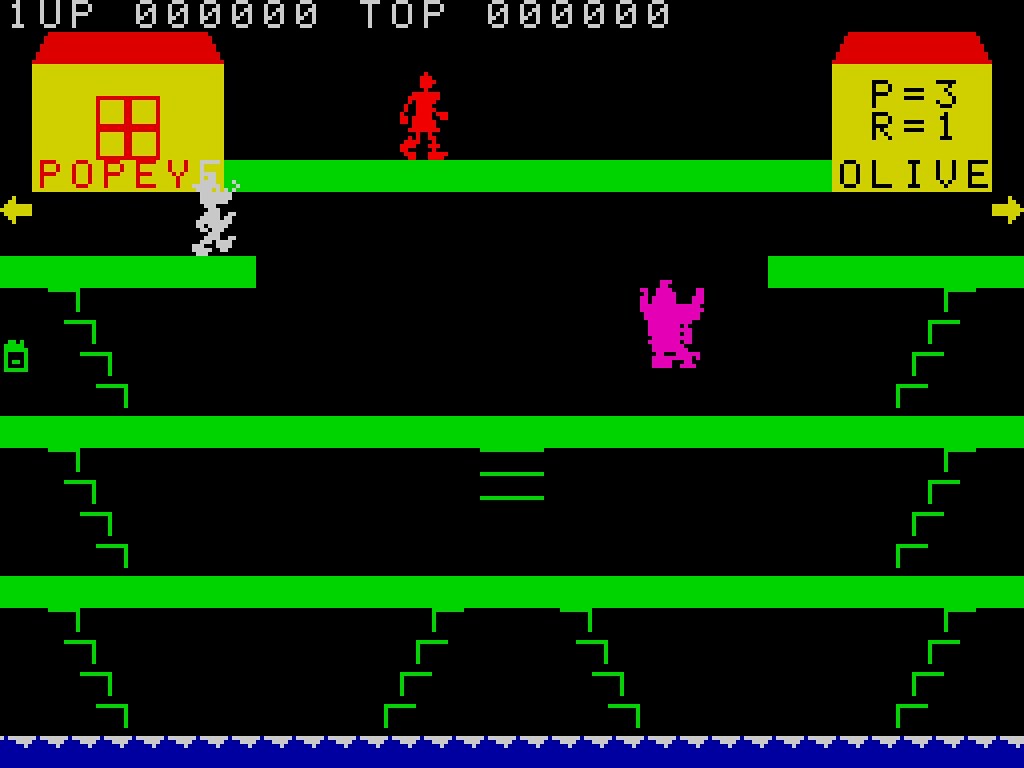This image is a still from a Popeye-themed video game featuring classic Atari-style graphics. The background is solid black. At the top of the screen, white digital print reads "1UP 000000" and "TOP 000000," indicating that no score has been recorded yet. Prominently displayed in the game, there is a yellow block structure with a red roof, resembling a house, marked with the text "POPEY," and another labeled "Olive," alongside the phrases "P = 3" and "R = 1." The playfield consists of green horizontal bars extending across the screen. A red, spindly figure, likely representing Olive Oyl, walks on the upper green line, while a purple character floats in mid-air above the lower green bar. Below the house is a character, possibly Popeye, rendered in white with a muscular stance. The level design includes additional horizontal green ledges, steps descending toward the center, and a rudimentary ladder. At the bottom, there's a blue and white spiky field reminiscent of water. The gameplay area is populated by outlined characters, including a large pink blob-like creature.